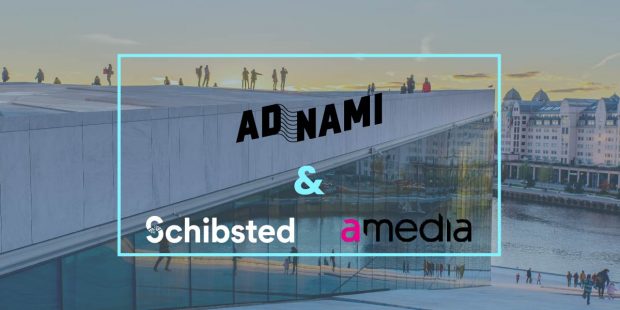The image, likely part of a slide presentation or advertisement, is in landscape orientation, approximately twice as wide as it is tall. The background depicts a modern cityscape during winter, with a prominent building on the left side that spans horizontally and is architecturally angled. This building features a large glass wall and people walking along its top, gazing into the horizon. Beneath this structure, people are heading towards a waterfront, implying access to a dock or riverfront. The scene includes snow-covered ground and a river flowing from right to left. In the far background, there are tall apartment buildings with blue roofs and beige facades, reminiscent of European cityscapes like Paris. Superimposed over the image, central text reads "ADNAMI & Schibsted A-Media," using a distinctive color scheme: "ADNAMI" in all black, "Schibsted" in white, and "A-Media" with a pink 'A' and black 'Media'. The overall color palette of the image is a grayish-blue, lending a serene atmosphere to the scene.